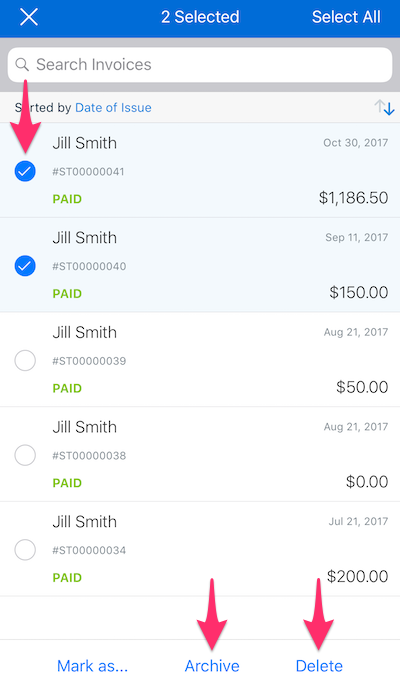In the image, there is a search interface designed to filter and sort invoices by their date of issue. At the top, two options are selected: "Select All" and "Search Invoices." An upward gray arrow and a blue downward arrow are present, indicating sorting options. 

Below, a sequence of transactions for Jill Smith is listed with detailed information:

1. **First Transaction**:
   - Date: October 30th, 2017
   - Invoice Number: ST00000041
   - Status: Paid
   - Amount: $1,186.50
   - Accompanied by a blue circle with a white checkmark for confirmation.

2. **Second Transaction**:
   - Date: October 30th, 2017
   - Invoice Number: ST00000040
   - Status: Paid
   - Amount: $150.00
   - Also marked with a blue circle and white checkmark.

3. **Third Transaction**:
   - Date: October 30th, 2017
   - Invoice Number: ST00000039
   - Status: Paid
   - Amount: $50.00
   - Displayed with a blue circle and white checkmark.

4. **Fourth Transaction**:
   - Date: October 30th, 2017
   - Invoice Number: ST00000038
   - Status: Paid
   - Amount: $0.00
   - Marked as paid with a blue circle and white checkmark.

5. **Fifth Transaction**:
   - Date: October 30th, 2017
   - Invoice Number: ST00000034
   - Status: Paid
   - Amount: $200.00
   - Similarly endorsed with a blue circle and white checkmark.

Towards the bottom of the interface, there are two prominent options in blue lettering: "Archive" and "Delete," accompanied by a red arrow pointing at both options. This indicates that users can choose to either archive or delete selected transactions.